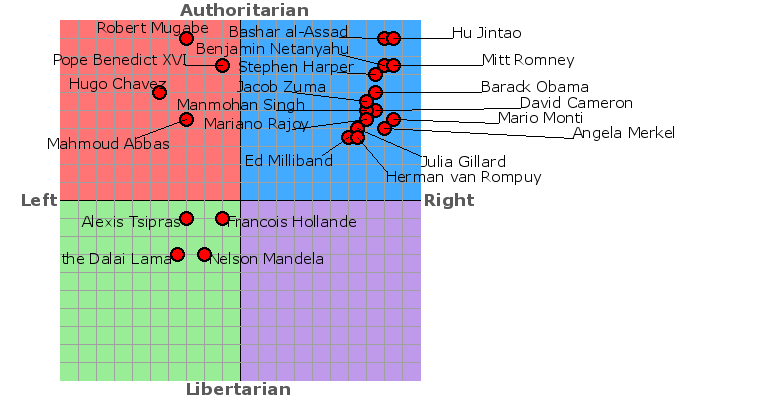The image displays a political spectrum chart designed to compare various individuals based on their political beliefs. The chart is divided into four quadrants with distinct colors: red for the top-left (left-wing authoritarian), green for the bottom-left (left-wing libertarian), blue for the top-right (right-wing authoritarian), and purple for the bottom-right (right-wing libertarian). 

The vertical axis ranges from "authoritarian" at the top to "libertarian" at the bottom, while the horizontal axis spans from "left" on the left side to "right" on the right side. 

Each individual is represented by a red dot, connected to their name through lines. For instance, Nelson Mandela's dot is positioned in the green quadrant, indicating that he is both left-wing and libertarian. Hugo Chavez's dot is located in the red quadrant, characterizing him as a left-wing authoritarian. Meanwhile, Barack Obama's dot falls in the blue quadrant, identifying him as a right-wing authoritarian.

This detailed political spectrum chart offers a comprehensive visual representation of where famous political figures are placed based on their ideological stances.